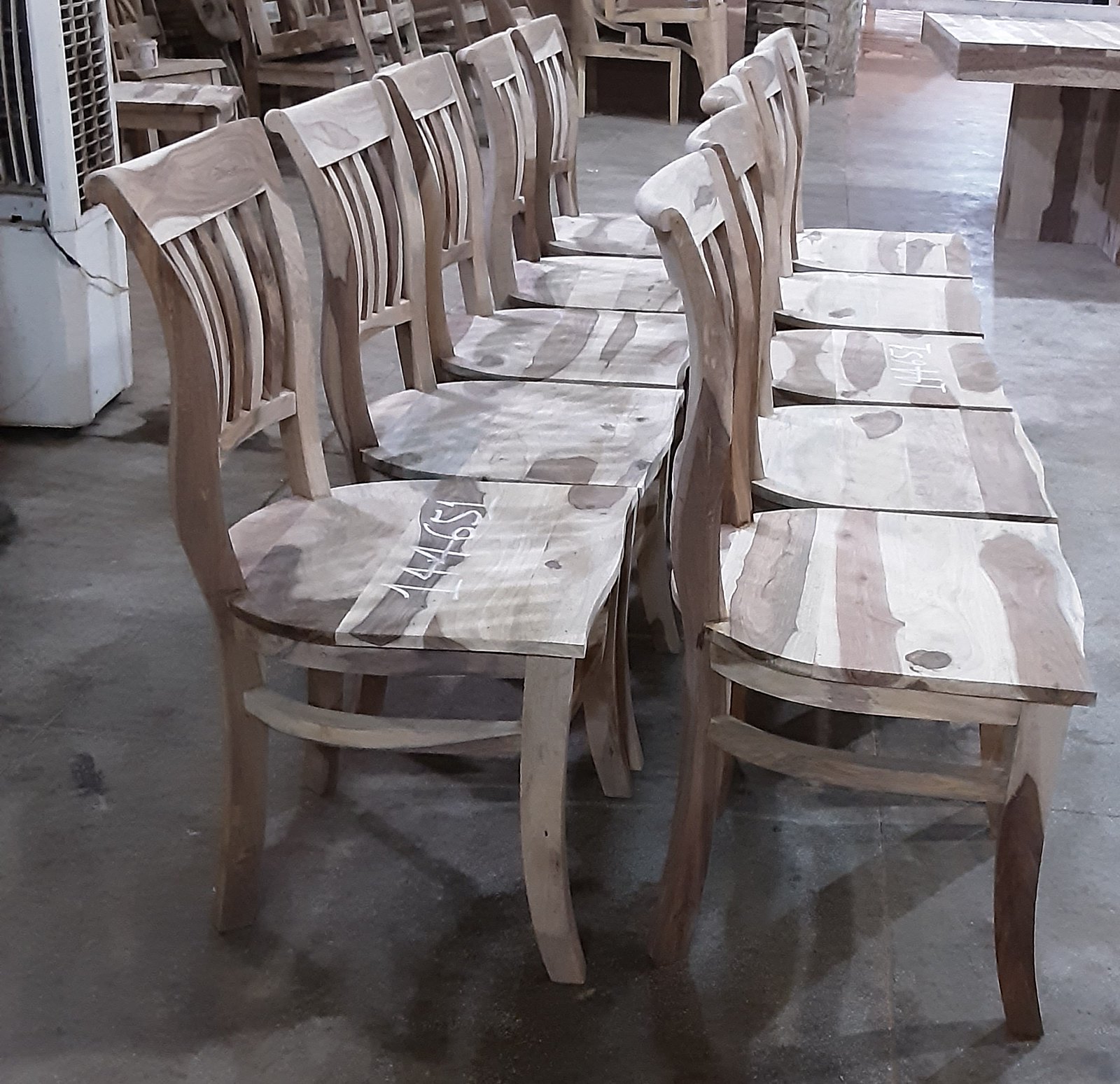The image depicts an industrial woodshop setting with a concrete floor. Dominating the foreground, ten unfinished wooden chairs are arranged in two rows of five, positioned side by side and touching each other. Each chair features a lumbar-supporting back panel and a shield-shaped seat for sitting. One chair stands out with the number "144651" written in white ink on its seat, potentially indicating a lot number. In the background, a workbench with a distinct wood grain pattern of light and dark colors can be seen, along with tables and chairs. The upper right corner of the image reveals a pallet sitting on something, while the upper left corner features a white piece of machinery with a vent, possibly an industrial air conditioning unit. The overall scene suggests that the chairs are either in the process of construction or awaiting finishing touches such as painting or varnishing.